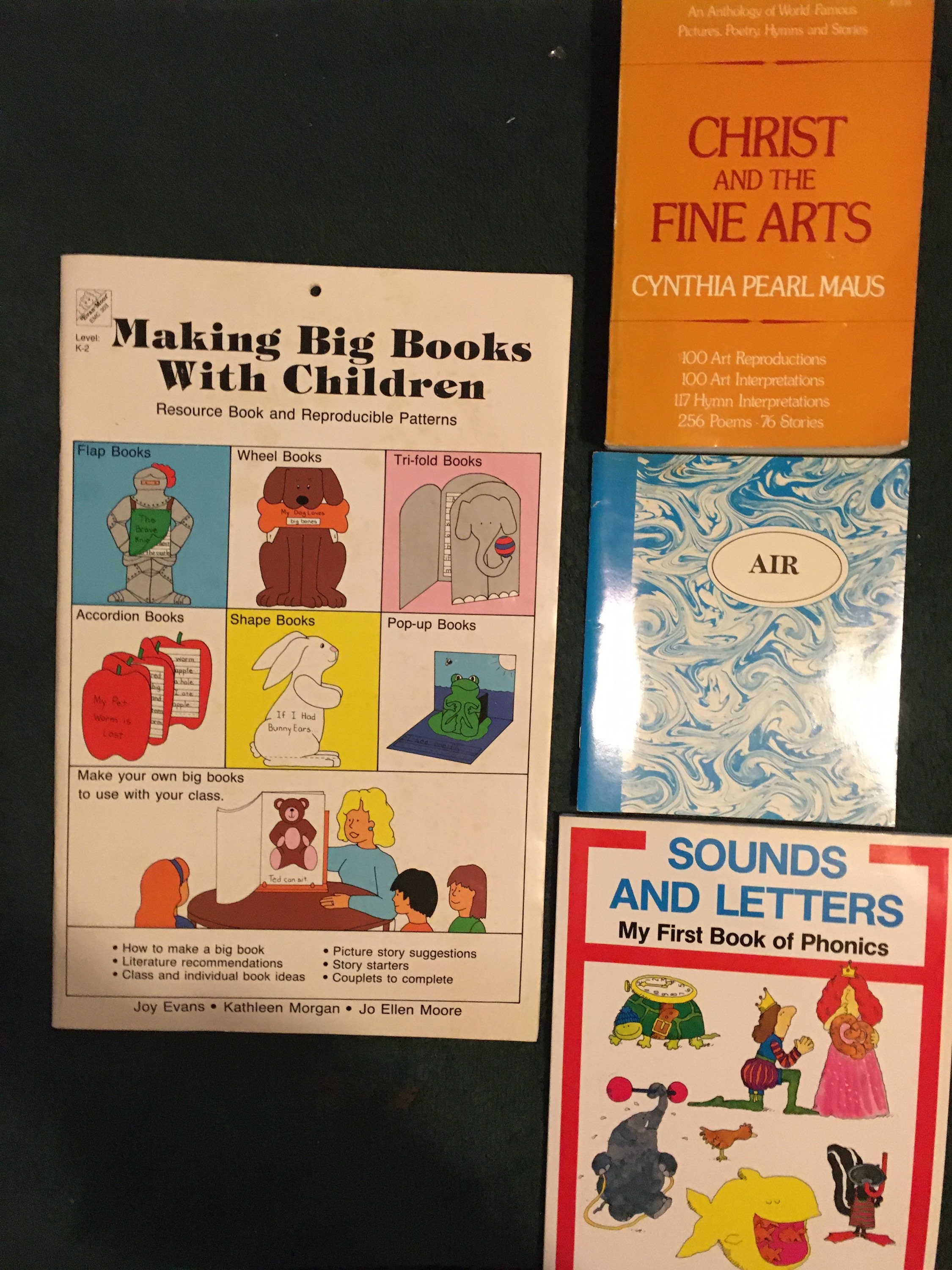The image showcases a display of educational books for children, neatly arranged on a black surface. On the left side, prominently featured, is "Making Big Books with Children: Resource Book and Reproducible Patterns," which is a large book with a white cover showing various patterns for creating accordion, flat, wheel, shape, pop-up, and trifold books. On the top right, an orange book titled "Christ and the Fine Arts" by Cynthia Pearl Maus is displayed, highlighting its rich content of 100 art reproductions, art and hymn interpretations, 256 poems, and 76 stories. Below it, there is a small, personal notebook labeled "Air" with a swirly blue and white background. At the bottom right, "Sounds and Letters: My First Book of Phonics" features a white cover adorned with illustrations of a prince, princess, and various animals—perfect for engaging a child in early reading skills.